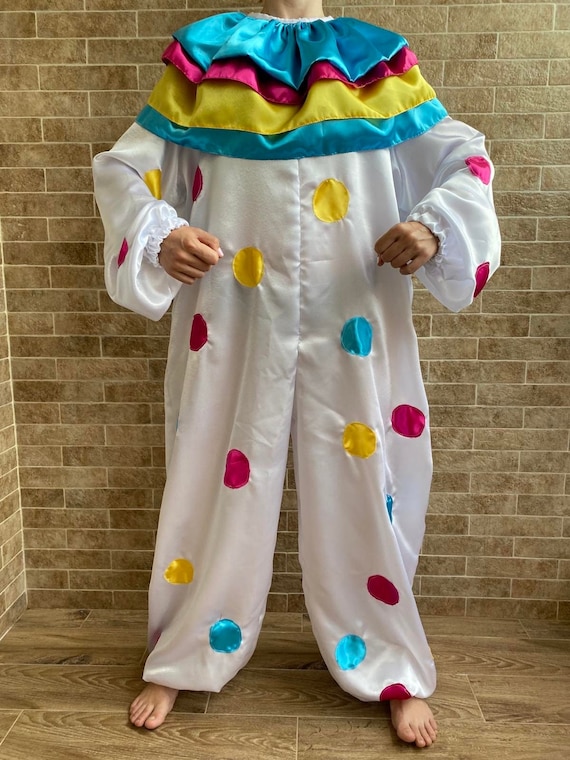In this photograph, a person dressed in a handmade clown costume stands against a tan brick wall on a light wooden floor. The clown outfit consists of a white, billowy, long-sleeve jumpsuit adorned with scattered multicolored polka dots in yellow, fuchsia, and turquoise blue. Around the neck, a large ruffled collar is layered with shiny, satin-like material in tiers of aquamarine blue at the top, followed by hot pink, yellow, and another layer of aquamarine blue. The person’s arms are bent at the elbows, with hands clenched into fists in front of their chest, revealing a distinctly animate presence despite the absence of their head in the frame. Additionally, their bare feet are visible at the bottom of the image, further emphasizing the human form within the clown costume.